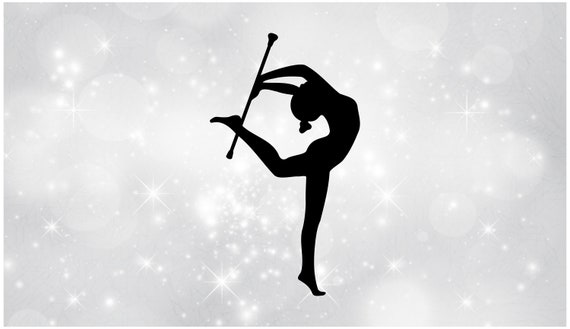The image is a monochromatic silhouette of a little girl, or possibly a woman, performing an intricate dance maneuver with a baton. Set against a grayish-white background adorned with bright, sparkling stars, the dancer exhibits remarkable flexibility and grace. She is depicted standing en pointe on one tiptoe, with her body arched backward so dramatically that her head nearly meets her uplifted leg, forming a U-shape. Her arms extend behind her, holding the baton in such a way that it crosses her body, enhancing the circular form. Her hair is styled meticulously into a bun at the back of her head. Despite the starry embellishments, the background remains a subtle contrast to the vivid expression of the dancer in silhouette, emphasizing her skill and poise in this ballet-like pose.